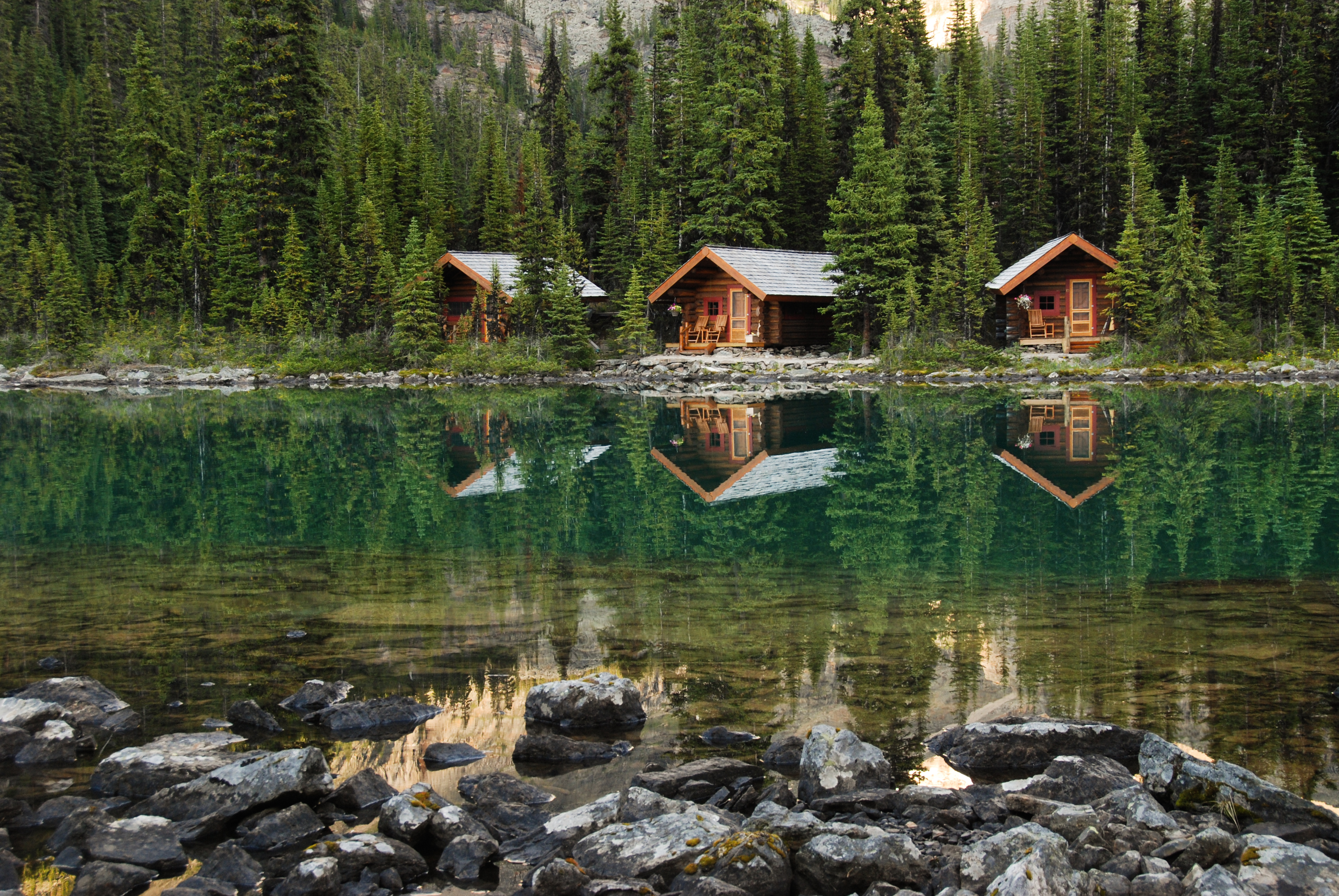The image captures a serene lakeside scene featuring three charming wooden cabins nestled amidst a dense, dark green coniferous forest. These rustic cabins, constructed from reddish-brown timber, stand along the far shore of a tranquil lake, likely in a mountainous region. Their lighter-colored tin roofs subtly contrast with the rich wood tones. 

In the foreground, smooth rocks and shallow water lead to the emerald-green lake, which mirrors the cabins and the surrounding pine or cypress trees with remarkable clarity. The water's jade hue is a reflection of the lush greenery enveloping the area. 

In the background, distant slopes, dusted with a whitish hue, suggest highlands or mountains rising behind the idyllic scene. The soft, even lighting indicates the photo was taken either in the gentle glow of early morning or during the calm light of late afternoon, enhancing the peaceful ambiance of this secluded, forested retreat.